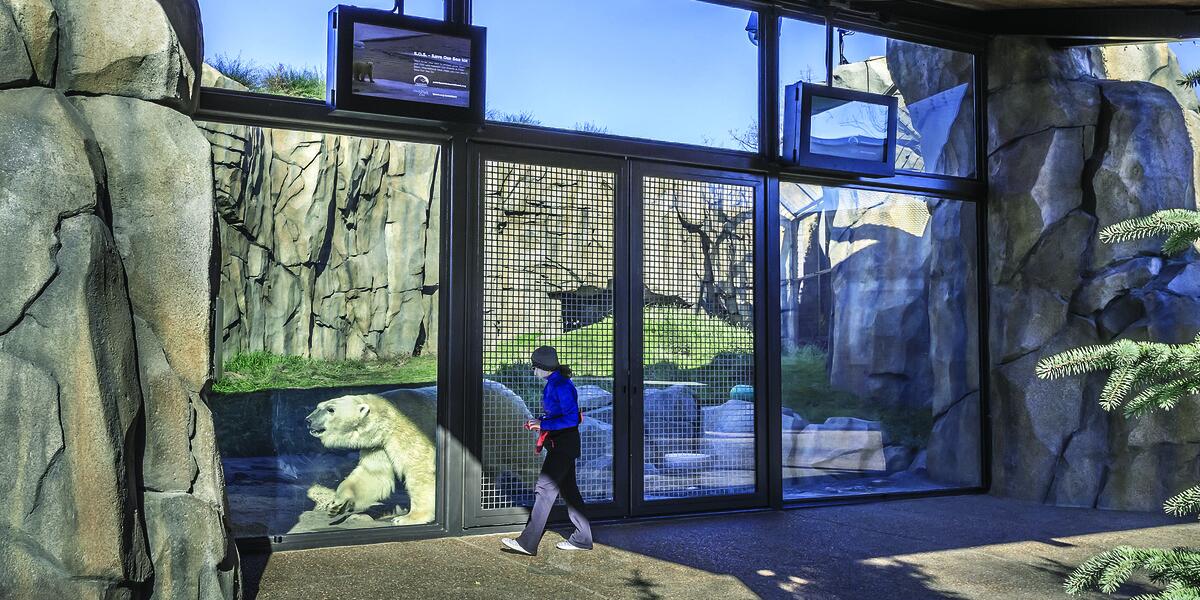The image depicts a detailed zoo exhibit featuring a polar bear in an enclosed habitat. The polar bear is positioned near the middle of the scene, pressing its paw against a floor-to-ceiling glass barrier that separates it from its observers. The enclosure is fortified with mesh wire and surrounded by towering rock formations on both the left and right sides. Grass patches and chunks of ice are scattered within the enclosure, creating a semblance of the bear's natural habitat. The bottom of the image shows a cement pavement, leading to the glass wall that entirely secures the polar bear's area.

Two TV monitors are mounted above the glass barrier, presumably displaying informational content about the polar bear. In the foreground, outside the enclosure, a person dressed warmly for the morning chill – wearing a blue coat, black pants, beanie, gloves, and a face mask – is walking towards the glass barrier, seemingly captivated by the majestic animal on the other side. Green pine trees further adorn the scene, emphasizing the constructed yet immersive environment of the exhibit.